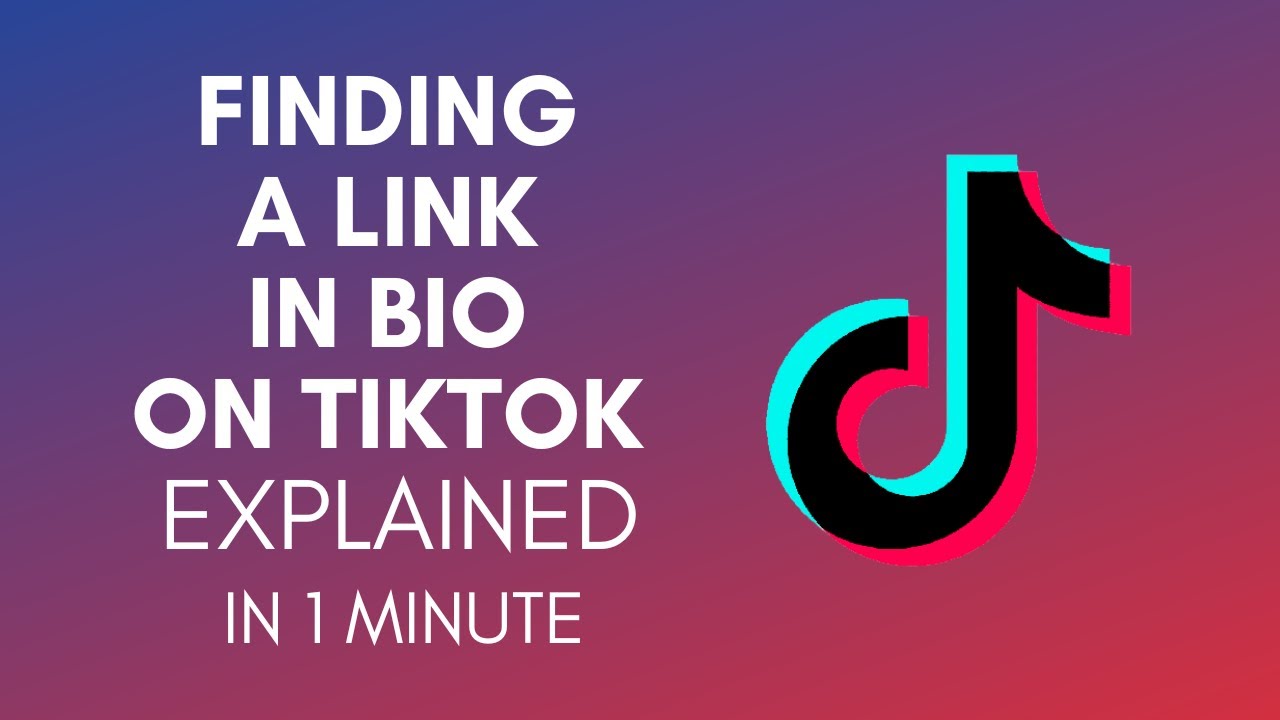The illustration vividly depicts the process of locating a link in a TikTok bio, explained concisely in one minute. The background features a gradient palette, transitioning seamlessly from a serene blue at the top, through a rich purple in the middle, to a vibrant pink at the bottom right. On the left side, blue and pink hues layer over each other, creating a dynamic and colorful display. Accompanying the vibrant backdrop, two overlaying black TikTok symbols are located to the right, adding a distinctive touch to the composition. The caption prominently displays the text, “Finding a Link in Bio on TikTok Explained in One Minute,” effectively encapsulating the essence of the visual content.